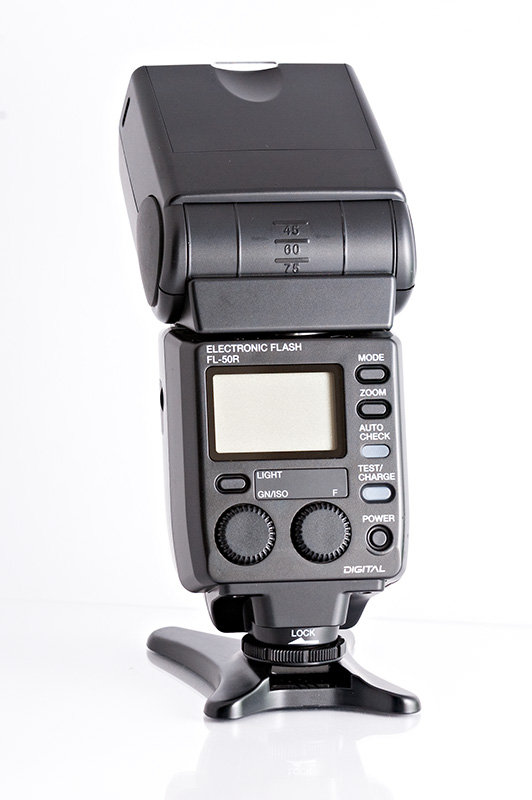The image features a detailed view of an electronic flash unit, specifically the FL-50R model, designed for professional photographers. It is set against a pure white background and mounted on a small, black X-shaped stand. The flash unit itself is dark gray and has a sophisticated control panel on its back side, indicating its high functionality and adjustability.

The control panel includes a digital display screen with a tan background and is surrounded by several buttons with extensive white labeling. To the right of the display, there is a column of four oval, cylinder-shaped horizontal buttons labeled "mode," "zoom," "auto check," and "test charge." A small round button is situated in the corner below these. On the left side below the display, there are two textured, round push buttons. Above these, the unit has indicators for settings such as GN, ISO, and F-stop values.

The text "electronic flash FL-50R" is prominently displayed above the digital screen in white lettering. Additionally, the lower right corner of the control panel features the word "digital." The upper portion of the flash unit comprises a cylindrical mechanism with angle markers, allowing the flash to tilt and adjust angles accurately. At the top, a cylindrical part labeled "lock" can be seen, indicating it may secure certain adjustments or attachments.

The overall design shows this equipment is highly versatile and suitable for various photographic needs, making it an essential tool for digital camera users.